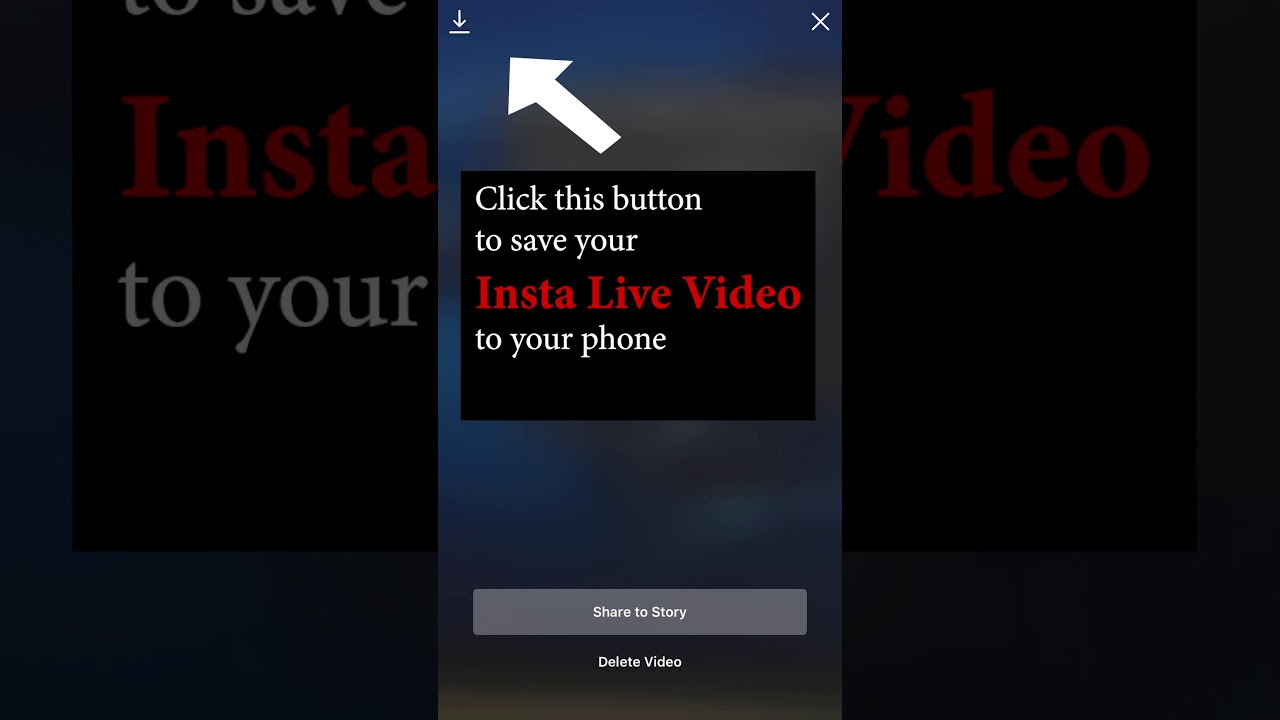This image features an instructional phone screen with a predominantly black background and raindrop-like elements scattered across it. Central to the image is a rectangular dialog box framed by a thin white border. In the upper right-hand corner of this box, there is a white "X" icon, indicating an option to close the dialog. On the upper left-hand corner, there's a download arrow icon, emphasized by a large white arrow pointing toward it.

Inside the box, the same black background with raindrop patterns is visible, making the elements inside stand out. Text within the box reads, "Click this button to save your Insta Live video to your phone." Below this instruction, there are two options: "Share to Story" and "Delete Video." This screen appears to be from a mobile interface of Instagram, allowing the user to manage their Instagram Live video by either saving it to their device, sharing it to their Instagram Story, or deleting it.